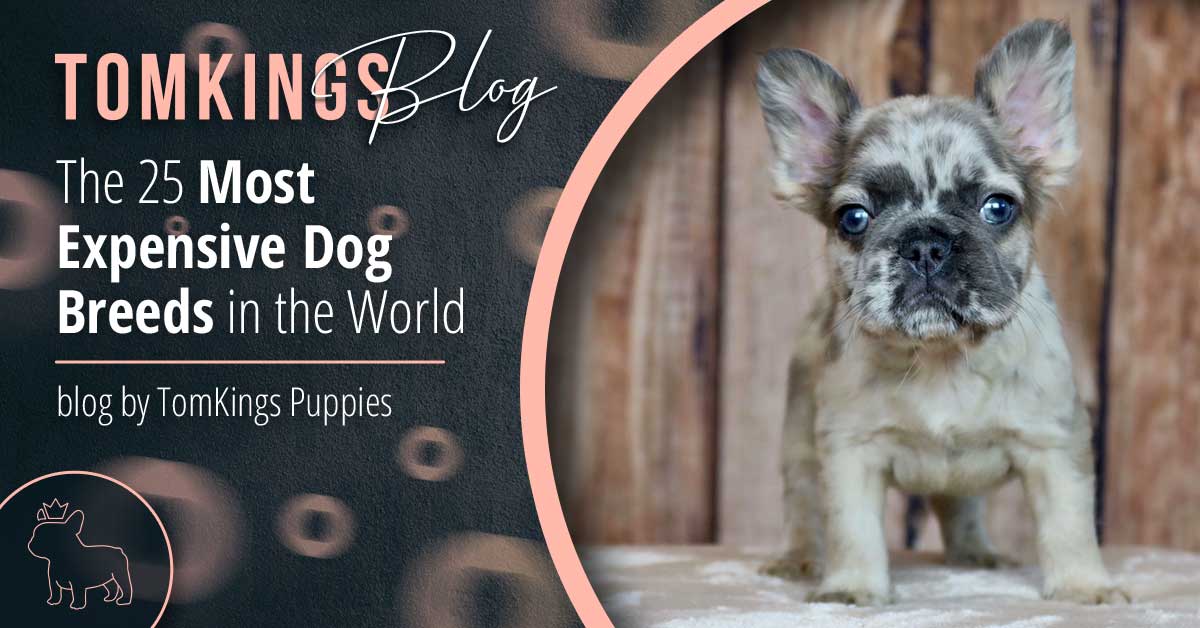The image is a flyer prominently featuring a small, brown and white dog with a distinctive pug-like face, perky ears, and hints of pink on its ears, standing on a white surface against a background of vertical wooden slats. The text on the flyer reads "Tom King's Blog" in a pink, all-caps font for "Tom King's" and a white, cursive script for "Blog," with only the "B" capitalized. Below that, in bold and thin white text, is the title "The 25 Most Expensive Dog Breeds in the World." A thin pink divider line separates this text from the subheading, "Blog by Tom King's Puppies," also in thin white font. At the bottom left corner, there's a pink circle with an outlined image of a dog wearing a crown, which appears to be the logo for Tom King's Blog. On the right-hand side, there is a thick pink circle, partially cut off, accentuating the composition.